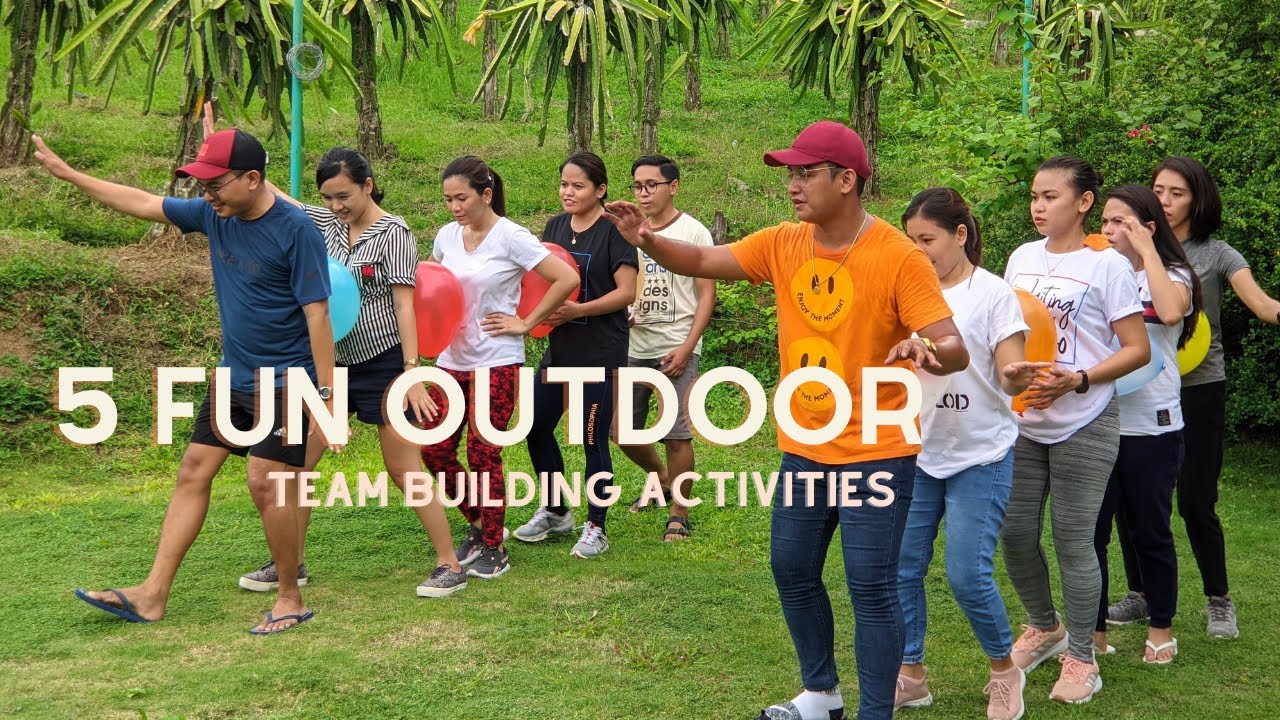The image appears to be a motivational poster or advertisement for team-building activities set in a tropical, Hawaiian-like setting. The background features lush greenery with palm trees and various plants. In the forefront, the central text reads "Five Fun Outdoor Team-Building Activities."

The scene captures two symmetrical groups, each consisting of five people standing in a line on a well-manicured grassy area. The participants are arranged in mirrored lines with mixed genders. The lead person in the line on the right wears an orange shirt and red cap, extending his arms outward as though engaging in the activity with enthusiasm. Similarly, the lead person in the left line dons a blue shirt, black shorts, and a red-and-black cap, also raising his arms skyward.

Behind these front leaders, the teammates in each line stand close together with four balloons strategically wedged between each pair, promoting a collaborative effort. The activity depicted evidently involves maintaining the balloons in place without letting them fall, fostering teamwork and coordination. The overall vibrant and energetic ambiance of the scene underscores the joyful and interactive nature of these outdoor team-building exercises.